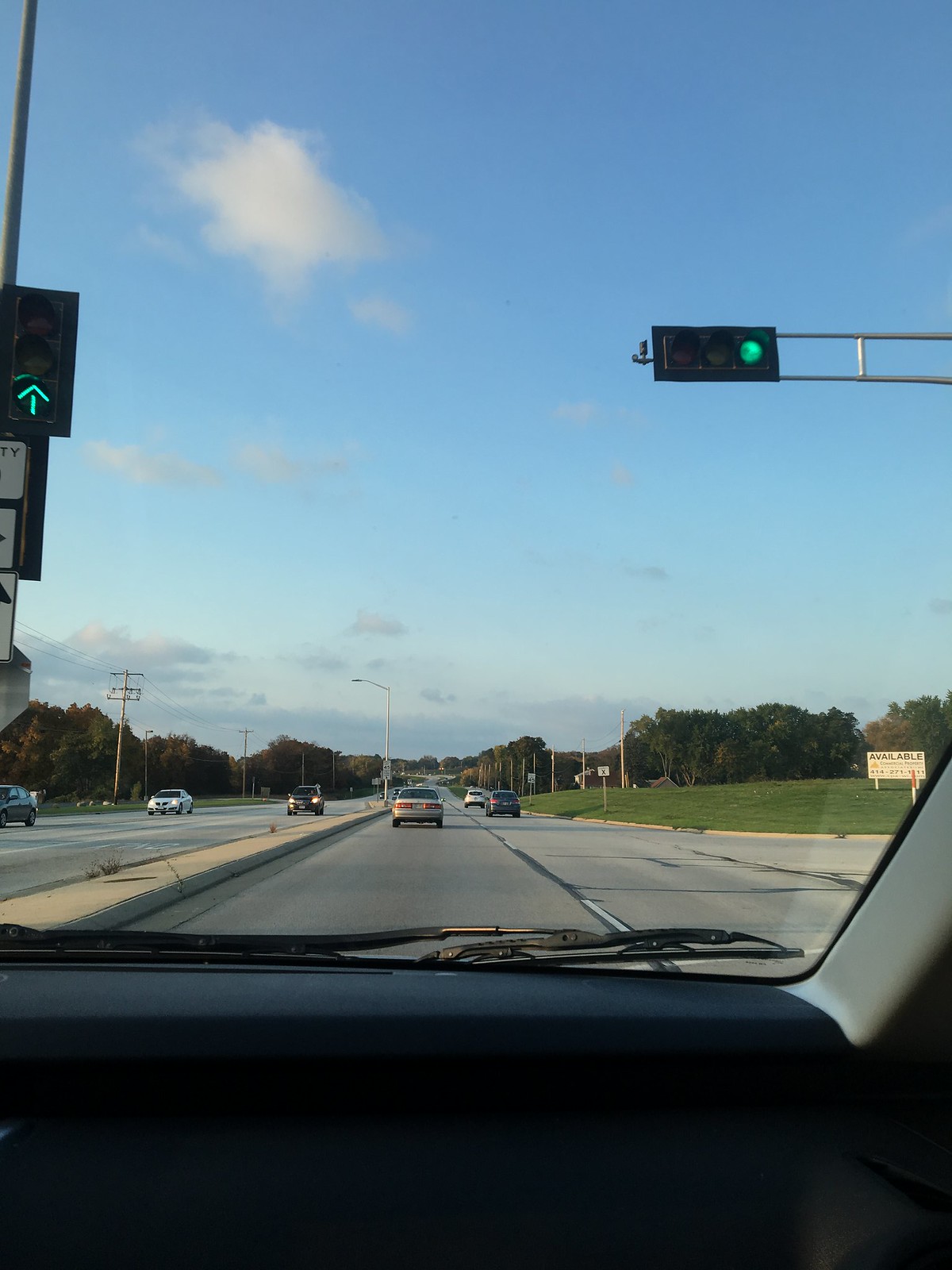Captured from inside a vehicle, likely on the passenger side, this photograph offers a view through the car's window. Dominating the scene is a green traffic light, mounted horizontally on a black fixture. The green light shines brightly, signalling for traffic to proceed. Beneath the traffic light, the road unfolds as a gravelly asphalt stretch, showing signs of black patch repairs. White lane markers are visible, delineating the traffic lanes. Off to the left, a median separates the opposing lanes of traffic. Ahead of the vehicle, a couple of cars can be seen with their brake lights illuminated, indicating they are coming to a stop or slowing down.